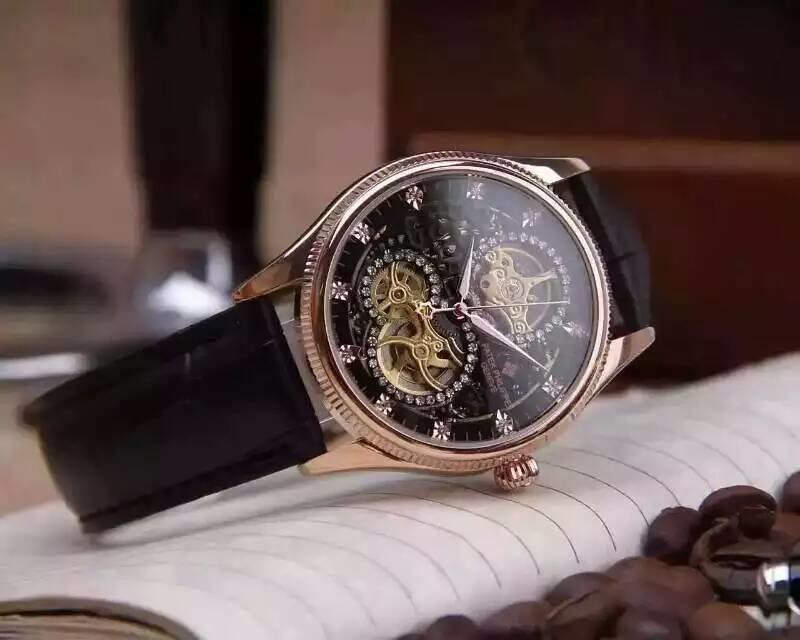The image showcases an elegant gentleman's wristwatch resting atop an open journal. The journal features lined paper, indicating it might be a diary or notebook. Adjacent to the journal, partially visible, are small brown beads, adding a subtle decorative element to the scene.

The wristwatch itself boasts a striking design with a black band and a gold-colored case. The dial is distinct, featuring leaf-like markers in place of traditional numerals to indicate the hours. The time displayed on the watch is 10:10. Notably, the watch reveals intricate internal mechanics, exposing the gears and movements, highlighted in gold with delicate rhinestones adorning a circular pattern around them. The second hand is in motion, capturing the essence of time in this sophisticated timepiece.